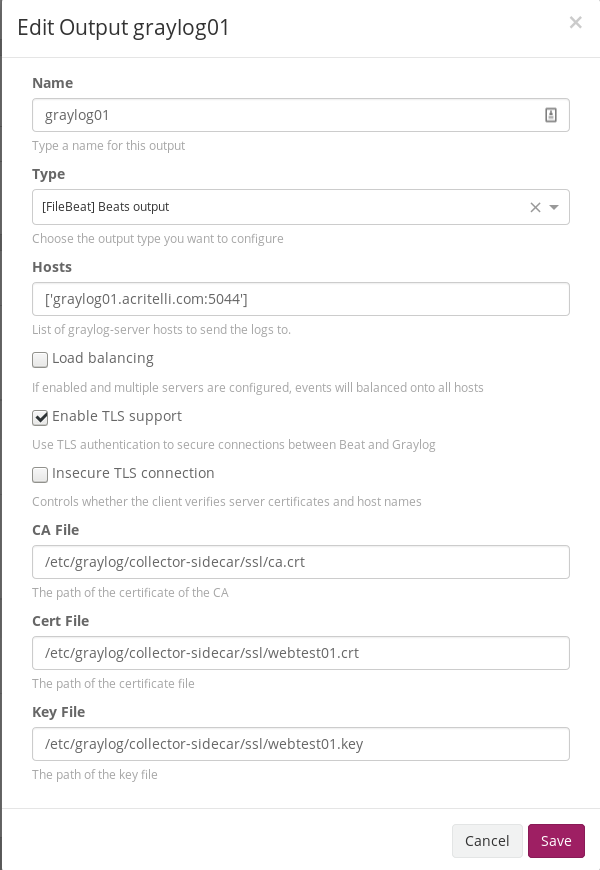This image depicts a screenshot taken from a mobile phone showing a configuration interface, identified by the title bar which reads "Edit Output: Graylog 01". Below the title, a faint gray line separates the header from the input fields.

The first section is labeled "Name," with an input box beneath it displaying "Graylog 01" alongside the instruction "Type a name for this output." The next section is marked "Type," featuring a dropdown menu that indicates the selected option as "Filebeat/Beats Output," followed by the guideline "Choose the output type you want to configure."

As we move further down the page, the "Host" section is visible, containing a field populated with various alphanumeric characters, intended to specify "List of Graylog server hosts to send the logs to." Below the host information, three options are available: "Load Balancing," "Enable TLS Support," and "Insecure TLS Connection." The "Enable TLS Support" checkbox has been selected.

Continuing downwards, additional fields for "CA File," "Cert File," and "Key File" are present, presumably for providing necessary security certificates and keys.

At the bottom of the interface, two buttons are visible: a gray "Cancel" button and a distinctive pinkish-burgundy "Save" button.